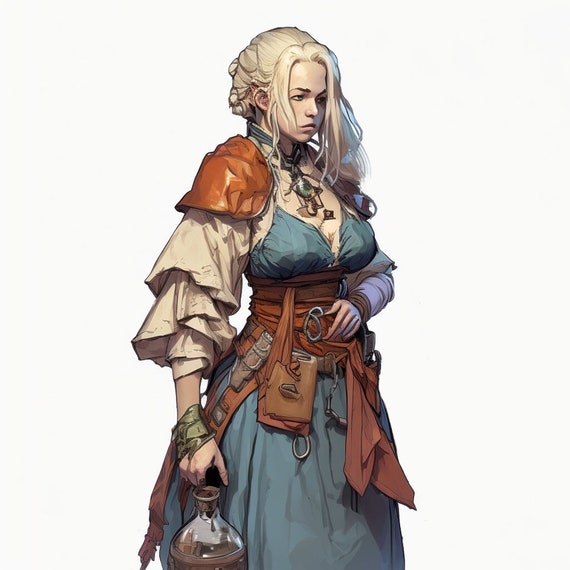This digitally rendered illustration, evocative of a drawing or painting, depicts a young woman reminiscent of a fantasy role-playing game character. The scene is set against a creamy, almost white background, spotlighting the woman as the central figure. She has very pale, almost white blonde hair, pulled back from her face except for some bangs hanging down. Her youthful appearance suggests she might be around 16 or 17 years of age. 

She is adorned in 19th-century styled attire, featuring a low-cut, light blue and white dress with cream-colored sleeves. Around her neck, she wears a large, bulky necklace with a prominent green jewel. Her waist is accentuated by a wide, brown belt or kit that wraps around several times, serving as a utility belt. Attached to this belt are numerous items, including pouches, possibly a leather pouch, a book, chains, and what appears to be a knife sheath. 

Her right shoulder is protected by a substantial leather pauldron, and similar protective leather wraps cover the backs of both her hands, adding to her adventurous appearance. In her right hand, which hangs down by her side, she holds a glass flask or jug. She gazes off to the right, exuding a sense of readiness and purpose.